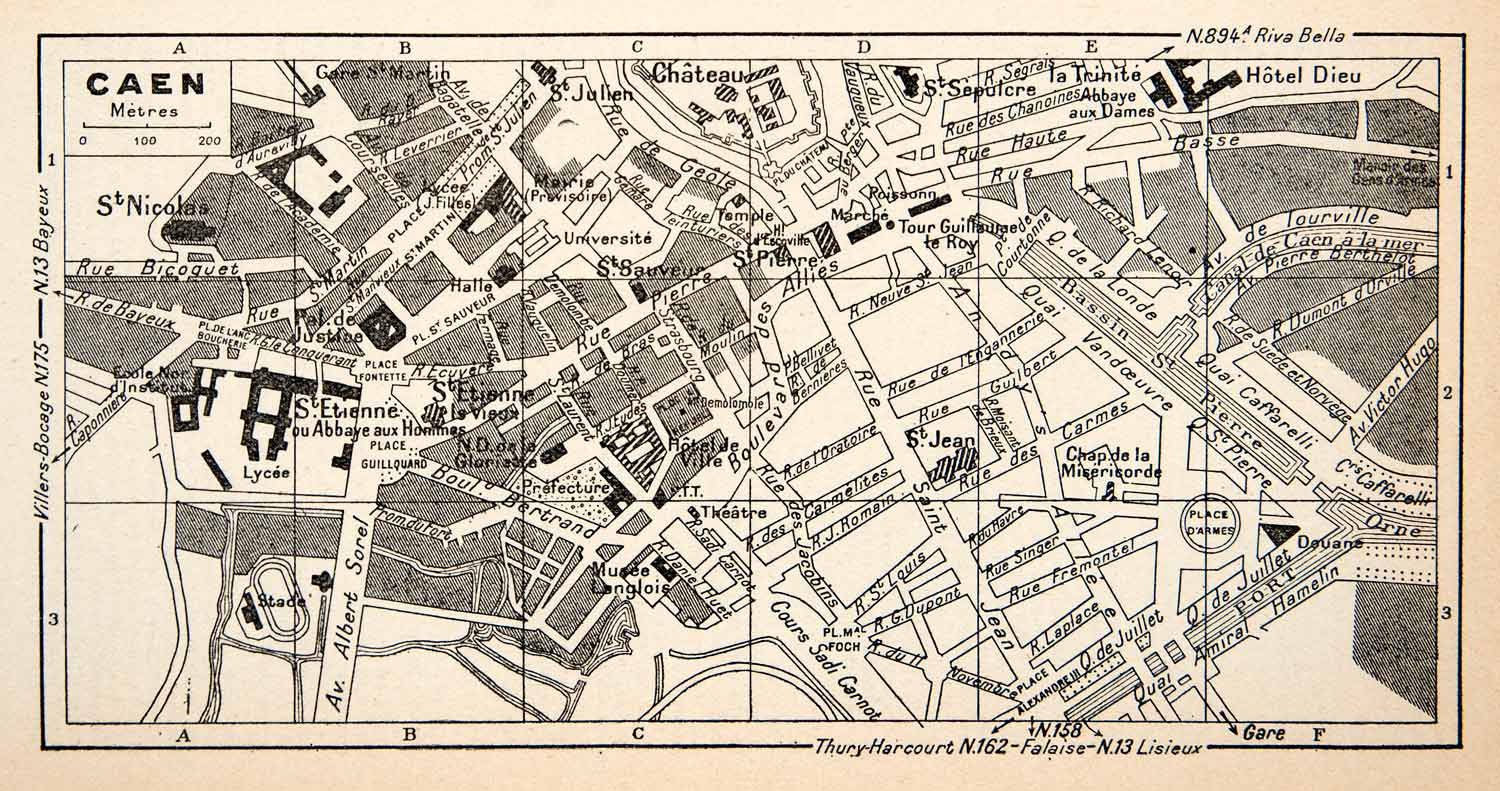This is an older, hand-drawn, black-and-white map of a city, likely in France, based on the French text and place names such as "Chap de la Misery Yard" and "Hotel Dieu" visible on the map. The map features a grid layout, with each street and landmark meticulously labeled in French, indicating the relative distances between them. The map's muted tones, achieved through black ink and gray shading, contribute to its antique appearance. Notable landmarks such as a stadium or a hotel are marked, further suggesting it is a detailed urban area. Text on the map includes names like Villers-Bocage and N175 to the left and Cayenne at the top, which might denote sections or surrounding areas of the depicted city. The map's overall condition and the color of the paper enhance its vintage feel, signifying it could be an old cartographic document.